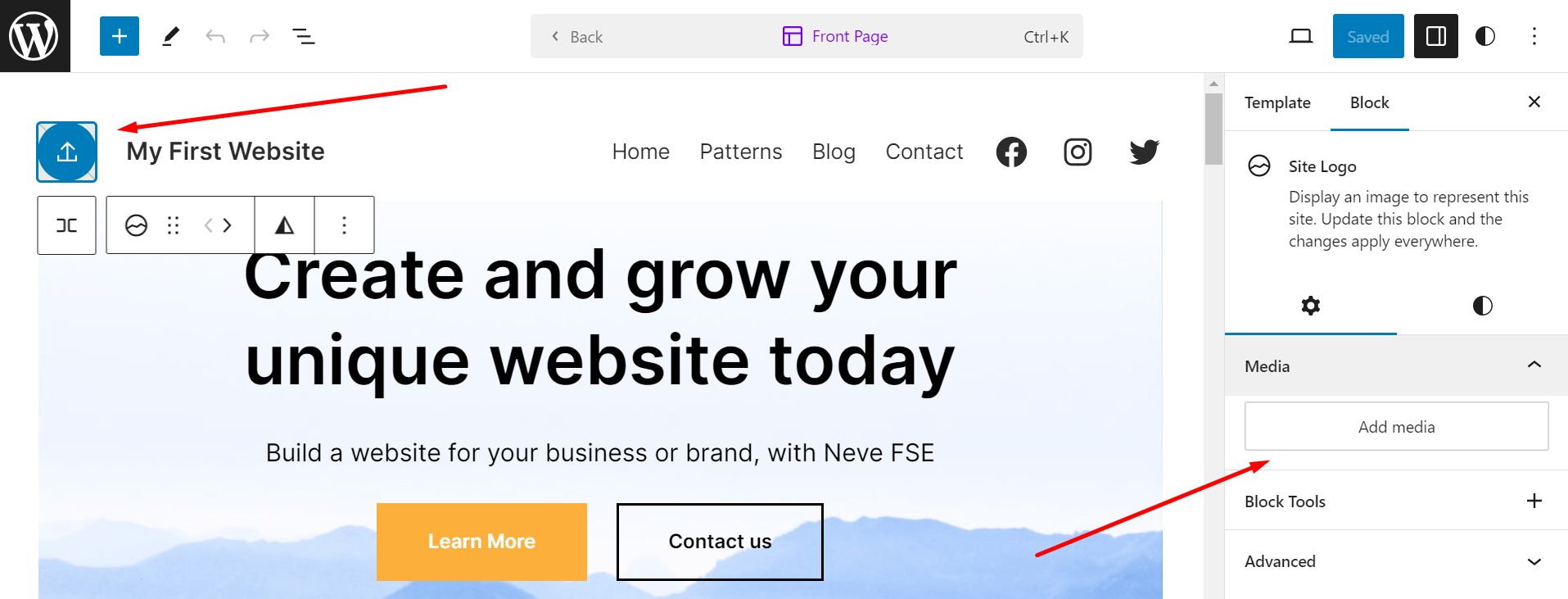### Descriptive Caption:

This image captures a detailed view of a web page. 

- **Top Left Corner**: A black square with a white "W" inside, outlined by a white circle.
- **To the right of the black square**: A white plus sign inside a blue box.
- **Further right**: A sequence of icons — a pen, a left arrow, a right arrow, and three diagonal horizontal lines.
- **To the right of the icon sequence**: A search bar with 'back' and a left arrow on the left side, 'front page' in the middle, and 'Ctrl + K' on the right side.

- **Below the icons on the left side**: A blue box with a white background that contains a blue circle and a download button. Next to this, the text "My First Website" is displayed with a red diagonal arrow pointing from the top of the image towards the download icon.

- **To the right of "My First Website"**: Blank space followed by menu items labeled "Home Page," "Patterns," "Blog," and "Contact." Social media icons (Facebook, Instagram, Twitter) are also displayed here.

- **Below the download section**: More icons, including:
  - An "X"
  - A circle
  - Two arrows pointing left and right
  - A dark black and white triangle
  - Three dotted lines

- **Main Content Area**: A picture with the text "Create and grow your unique website today" in black letters. Below this, the phrase "Build a website for your business or brand with Neve F SE" is displayed.

- **Background**: A blue sky with some blue mountains.

This detailed caption provides a comprehensive description of the web page layout and elements.